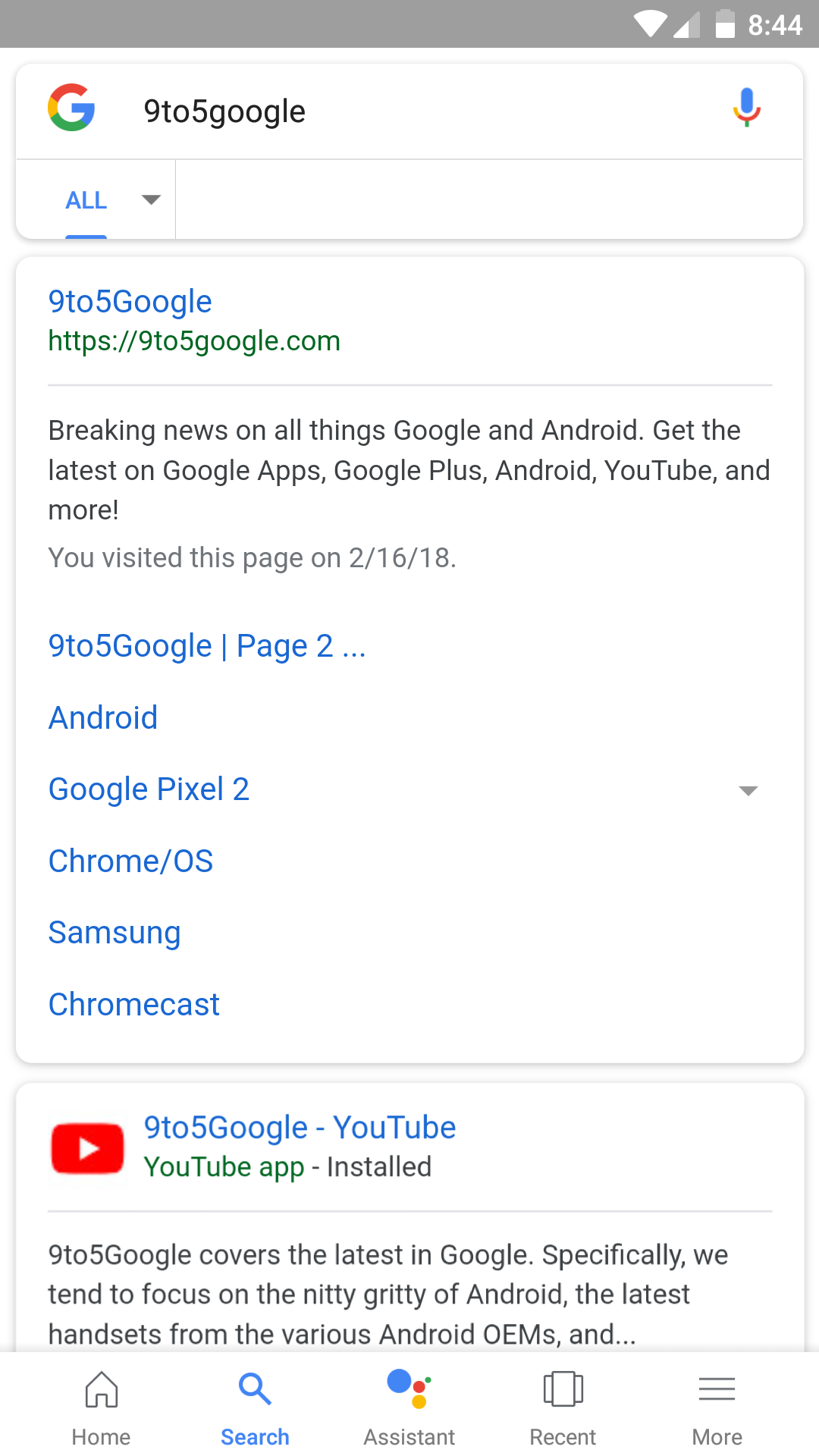The image showcases a cell phone screen displaying Google search results. The top right corner of the screen includes status icons: a wireless signal icon, a cellular connection icon, and a battery icon indicating a little more than half charge, accompanied by the time "8:44". The Google logo is prominently displayed on the far left at the top of the screen, with "9 to 5 Google" typed in the adjacent search box. Just below this, the navigation options include the word "All" next to a downward-pointing arrow.

The first search result is titled "9 to 5 Google" with the web address underneath. The description reads: "Breaking news in all things Google and Android. Get the latest on Google Apps, Google Plus, Android, YouTube, and more. You've visited this page on 2-16-18." Additional keywords listed include "Android, Google Pixel 2, Chrome OS, Samsung Chromecast."

The second search result features a rectangle with a red background and a play button on the left side, indicating a video link to "9 to 5 Google, YouTube." The description mentions that "YouTube app installed," followed by a brief outline of the content focus: "9 to 5 Google covers the latest in Google. Specifically, we tend to focus on the nitty gritty of Android, the latest handsets from the various Android OEMs, and..."

At the bottom of the screen, there are five icons representing different actions: a house (Home), a magnifying glass (Search), a few circles (Assistant), a page (Recent), and three horizontal lines (More). Below these icons, the respective labels read: "Home", "Search", "Assistant", "Recent", and "More".